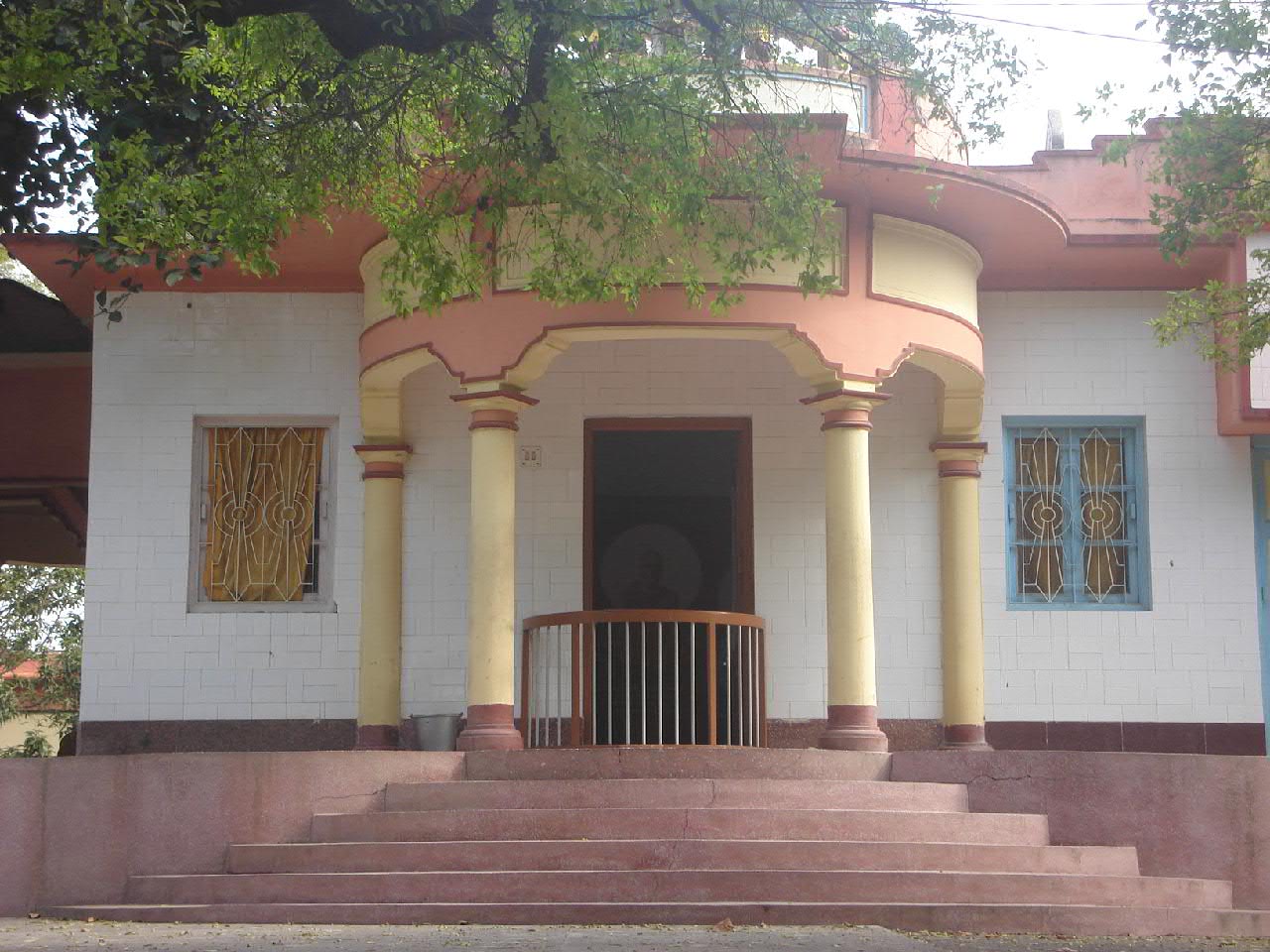This photo depicts the front of a small structure, possibly a Buddhist temple, set outdoors. The building features a distinctive design with a mix of dark pink, brownish, or clayish hues on the lower part of the exterior and porch area. There are approximately five concrete steps leading up to the entrance, flanked by a small, round gate with bars inside, providing a barricade. Four low columns, appearing somewhat dirty and yellowish, support a porch-like structure in front of the doorway. These columns share the same odd pinkish-brown color as the rest of the porch. 

The building's façade is made of white bricks or tiles, contributing to its distinct appearance. It includes two front windows fitted with protective bars against break-ins; interestingly, the window on the right features a blue tint, whereas the one on the left maintains a more wooden color. Overhead, tree branches laden with green leaves extend over the roof, adding a natural touch to the scene. To one side, there's a hint of signage, while more trees populate the background, framing the serene setting.